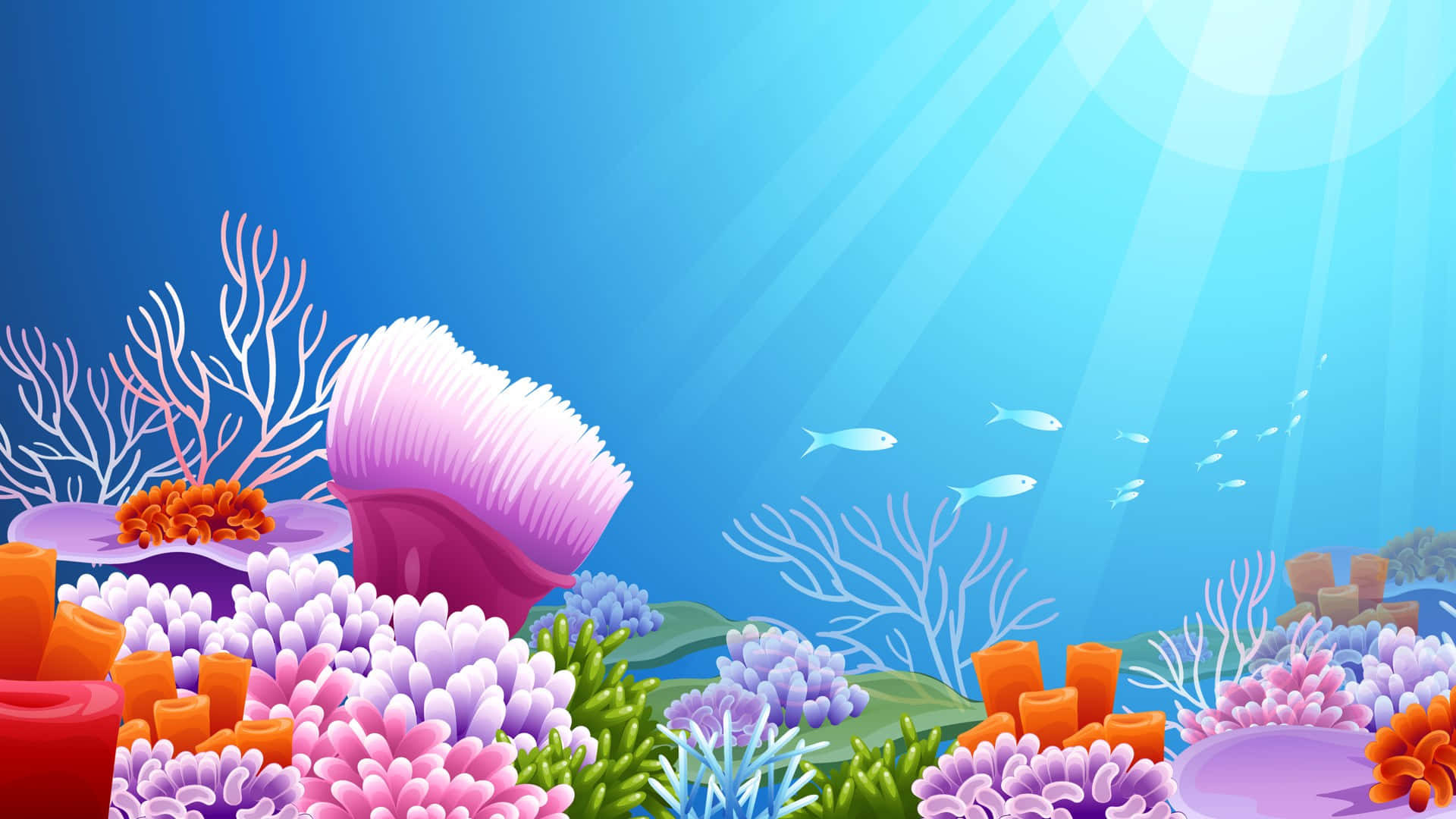This detailed digital illustration portrays a vibrant underwater scene bathed in shades of blue, transitioning from darker to lighter hues where sunlight penetrates the ocean surface. Rays of sunlight cascade from the upper right corner, illuminating a small school of blue and white fish swimming upwards. The foreground is teeming with life, dominated by an array of colorful corals and marine organisms. Various species of anemones in hues of orange, pink, and purple extend their tentacle-like structures, intermingled with green and blue sea cucumbers. Among the corals, which resemble rainbow-colored trees, are orange and red tube-like formations waving gently. The overall scene captures the bustling, colorful diversity of a coral reef ecosystem, showcasing the intricate beauty of life at the ocean's depths.